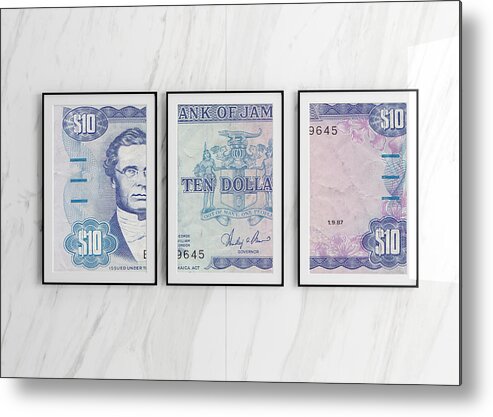This art piece features a $10 banknote from the Bank of Jamaica, meticulously cut into three segments and framed individually against a marble background, all enclosed in a thin black frame. The left frame showcases the front left portion of the bill, displaying "$10" at both the top and bottom and featuring a middle-aged, white man with glasses, short hair, thin lips, and formal attire—a white shirt and tuxedo. The center frame presents a portion of the banknote's text, partially revealing the inscription "Bank of Jamaica," along with some serial numbers and the beginning of the word "DOLLAR." Finally, the right frame contains the remaining segment of the banknote, including "$10" and additional serial numbers. The three frames collectively preserve the fragmented banknote, emphasizing its artistic transformation while retaining its original elements.